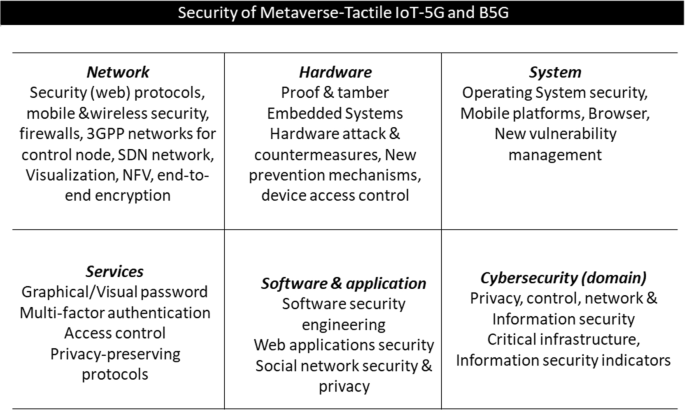Displayed on a plain white background with a black border at the top, the image showcases a detailed table entitled "Security of Metaverse, Tactile Internet of Things, 5G, and B5G." The table is structured into three sections and contains two rows, separated by thin black lines. The first row features columns labeled Network, Hardware, and System, while the second row includes Services, Software and Application, and Cyber Security Domain. 

Each section provides specific details on its area of focus:

- **Network**: Covers security web protocols, mobile and wireless security firewalls, 3GPP networks for a control node, STN network, visualization, NFC, and end-to-end encryption.
- **Hardware**: Discusses proof and tamper-resilient embedded systems, hardware tech countermeasures, new prevention mechanisms, and device access control.
- **System**: Includes operating system security, mobile platforms, browsers, and the need for new vulnerability management.

In the second row, the sections further elaborate:

- **Services**: Features topics like graphical visual passwords, multi-factor authentication, access control, and privacy-preserving protocols.
- **Software and Application**: Focuses on software security engineering, web application security, and social network security and privacy.
- **Cyber Security Domain**: Highlights privacy control, network and information security, critical infrastructure, and information security indicators.

The table outlines crucial aspects of cybersecurity across different domains and explains them in detail, making it a comprehensive resource for understanding security measures in advanced technology areas. The entire layout is predominantly in black and white.